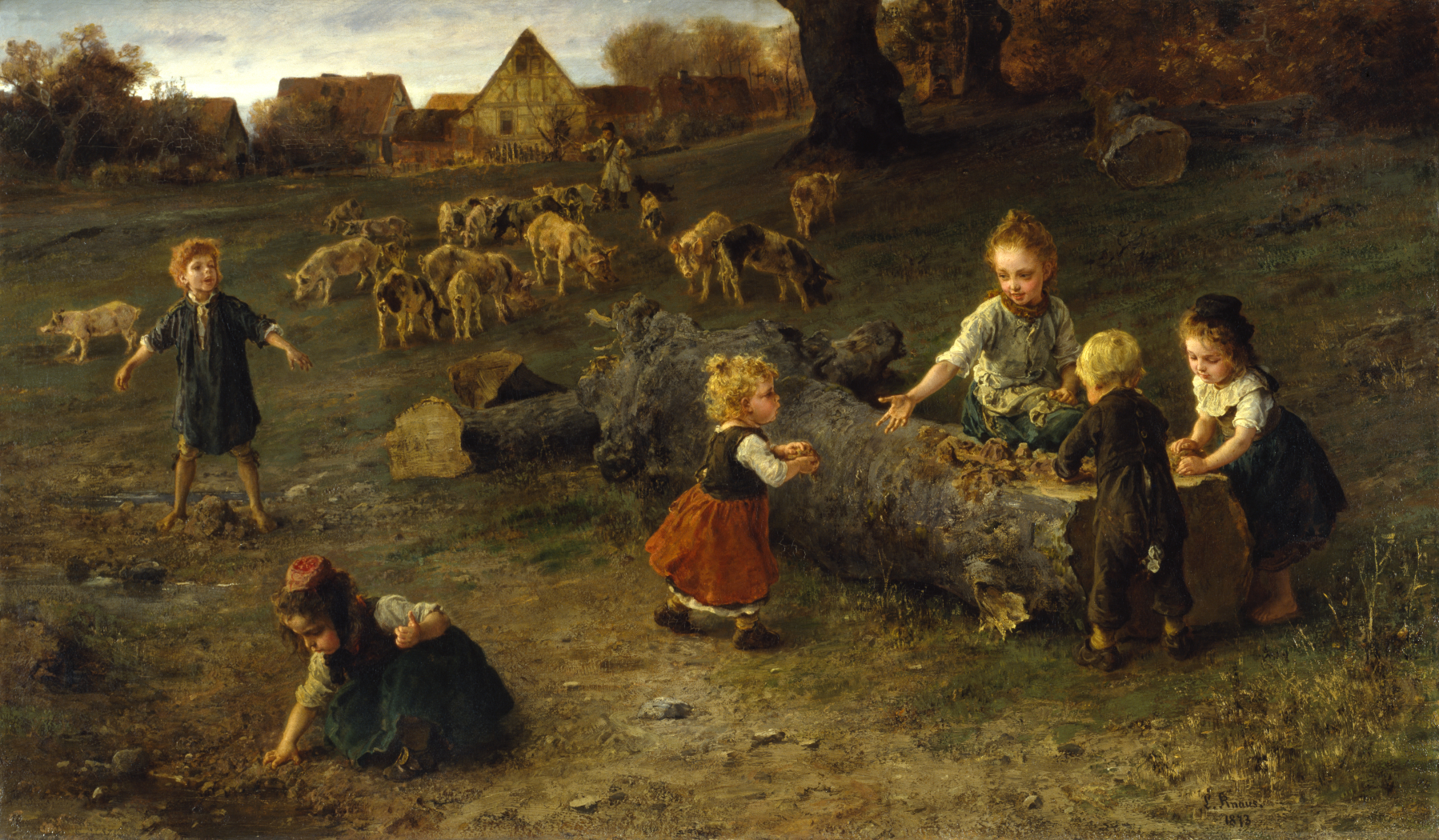The painting is a wide, rectangular canvas that captures a serene outdoor scene with a group of children and a rural village backdrop. This classical, realistic artwork is suffused with soft light and rich colors, portraying about four little girls and two boys, presumably siblings or neighbors, engaged in playful activities on a fallen log in the middle of a grassy field. The log, which has been flattened on top as if by an axe, serves as a makeshift table for the children who are making mud pies and small volcanoes. The children, dressed in simple play clothes, appear joyful and peaceful as they immerse themselves in their imaginative play.

To the left of the group, a little boy in a blue nightshirt stands with his arms outstretched, while in the foreground, a toddler girl bends over to pick up rocks. Another toddler girl, with blonde hair, walks towards the log, where an older blonde girl with her hair pulled back, sits facing away. On the other side of the log, a five-year-old girl joins in the play. Behind the children, a herd of pigs in off-white, gray, and black roam the field, tended by a shepherd. In the background, rows of small, greenish-gray and brown cottage-style homes are nestled among green trees tinged with brown, under a light blue sky dotted with white clouds. This idyllic scene evokes a sense of community among the rural villagers, who are likely livestock keepers and farmers.